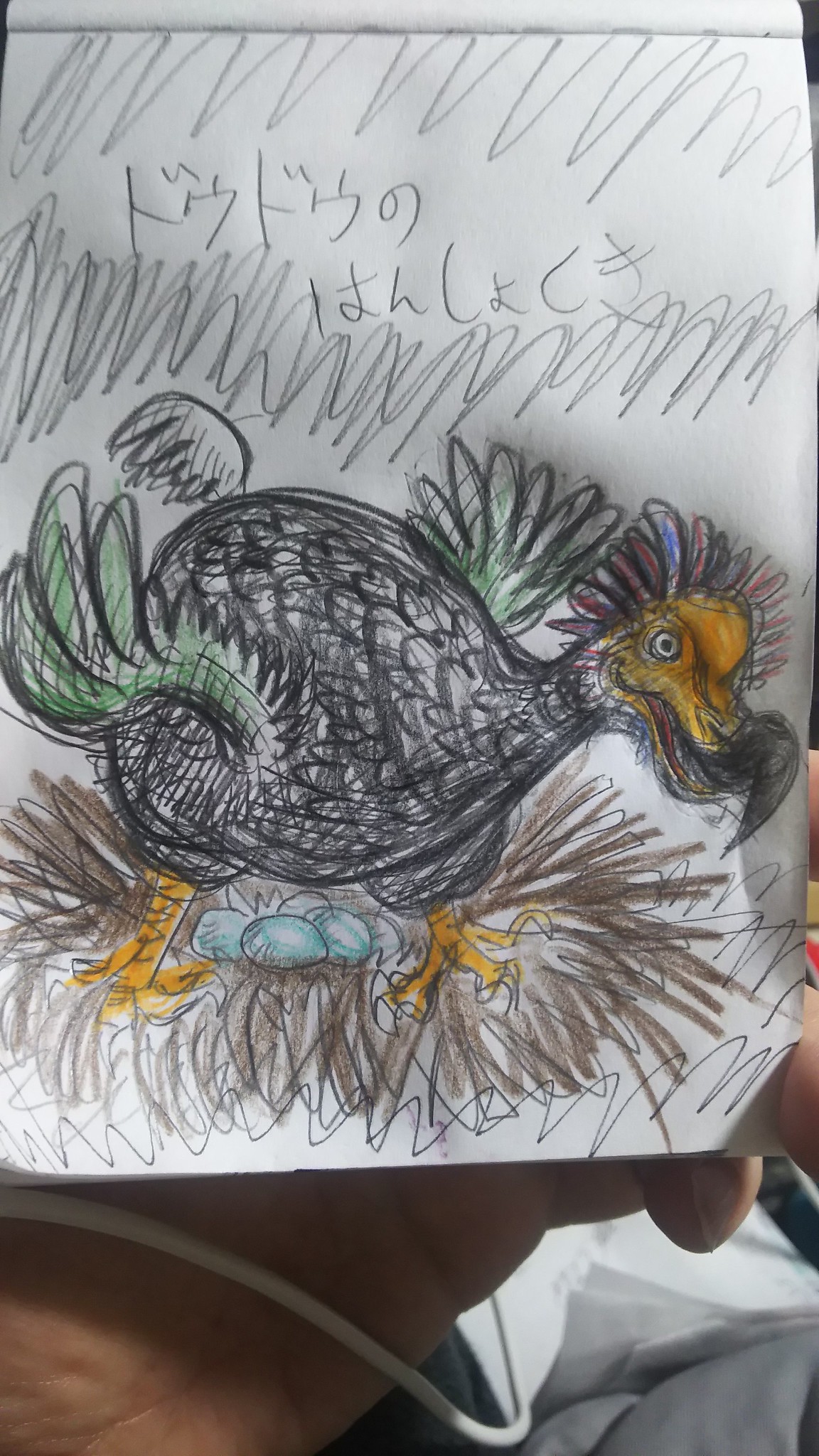A child's crayon drawing depicts a distinctive bird in profile, perched atop a nest containing five or six white and bluish eggs. The bird, which recalls the appearance of either a dodo or a rooster, has a dark tannish-orange head with a prominent white circular eye, green wings, and a body covered in black feathers. Its tail feathers extend to the left and head to the right, while a colorful plume with red, yellow, and blue feathers adorns the top of its head. The nest at the bottom of the image, formed by black or gray swirly lines, provides a base for the scene. Above the bird, pencil scribblings with wiggly lines stretch across the top of the paper, potentially forming an unreadable Asian script. Part of someone's hand holds up this image in the foreground, and a gray object with a white cord wraps around the hand in the bottom right corner. Though slightly blurry and stretched, the drawing captures a vivid and intricate scene.